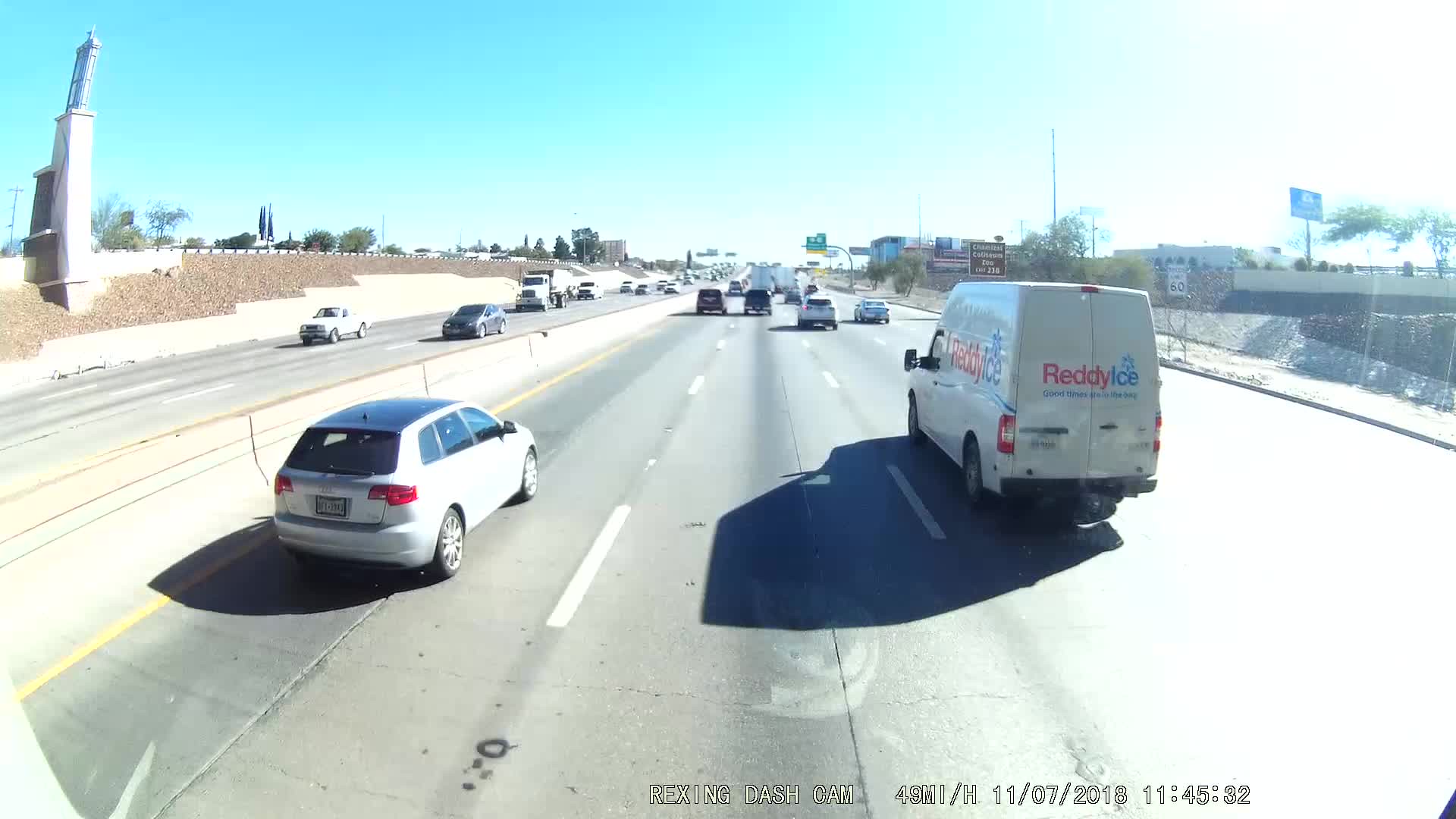The image captures a bustling street that closely resembles a highway, viewed from a slightly elevated, angled perspective as if taken from the vantage point of the middle lane. Dominating the foreground is a sturdy cement divider that runs through the highway, separating the traffic flow. Directly ahead, a white van can be seen navigating the lane, while to the left, a chromatic hatchback glimmers under the light. The background features an array of vehicles making their way down the road, suggesting a busy atmosphere. Prominently displayed along the highway are green exit signs that provide direction to motorists. Additionally, on the right side of the image, a brown sign is visible, likely indicating a point of interest or a service road exit. The photo captures the constant movement and directionality of urban traffic, encapsulating the organized chaos of roadway navigation.